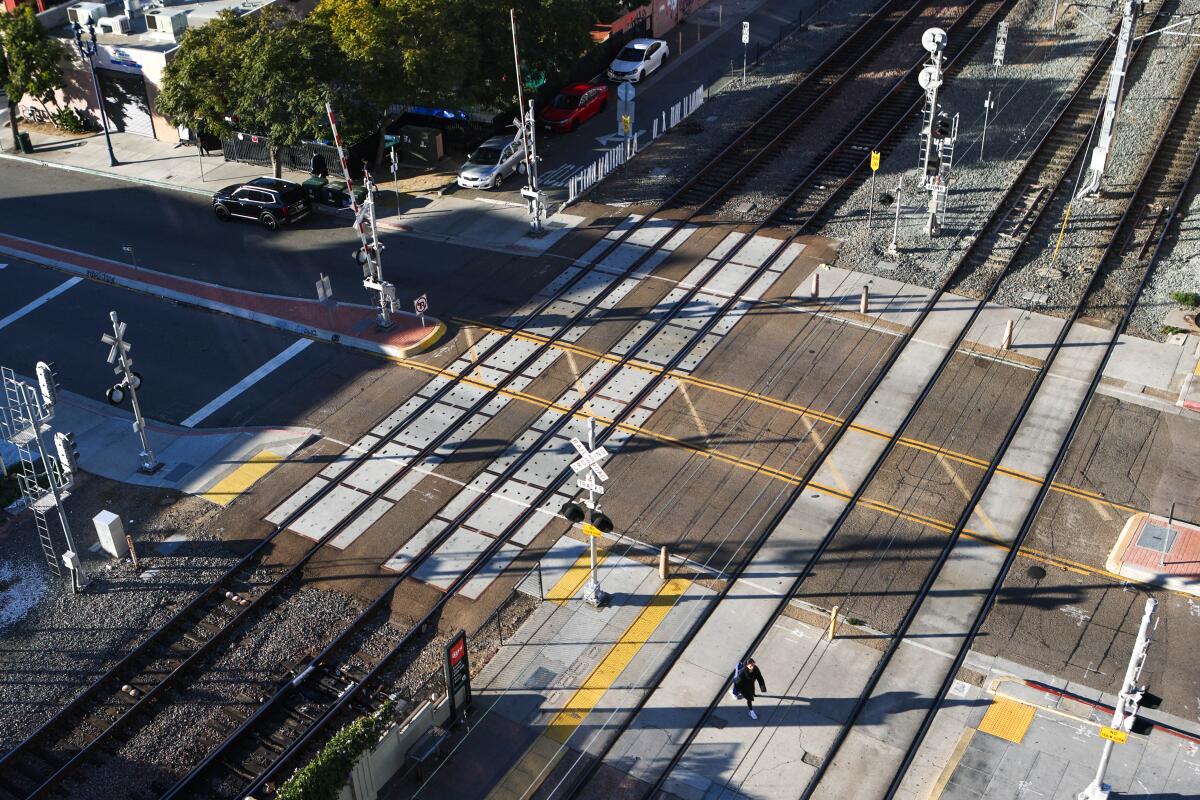This is a detailed, aerial color photograph of a large railroad crossing in a town, taken from a tall vantage point. The main feature is the intersection where a road with two double yellow lines crosses four sets of train tracks. The tracks run diagonally from the upper right to the lower left of the image, with a person walking across them in the bottom right corner. The crossing has standard railroad crossing signals, including flashing lights and arms that would lower to block traffic if a train were approaching, although no train is currently present. 

At the top left is a beige or white building partially obscured by green trees, with sidewalks in front and cars parked along the adjacent road. The parked cars are of various colors including black, silver, red, and white. The road and train tracks are also marked with various yellow and white indications to guide vehicles and pedestrians. There is a median dividing the road at the crossing point, and a gravel area can be seen at the top right of the photograph. The angle of the photograph provides a clear, diagonal view of the scene, emphasizing the scale and layout of the crossing area.